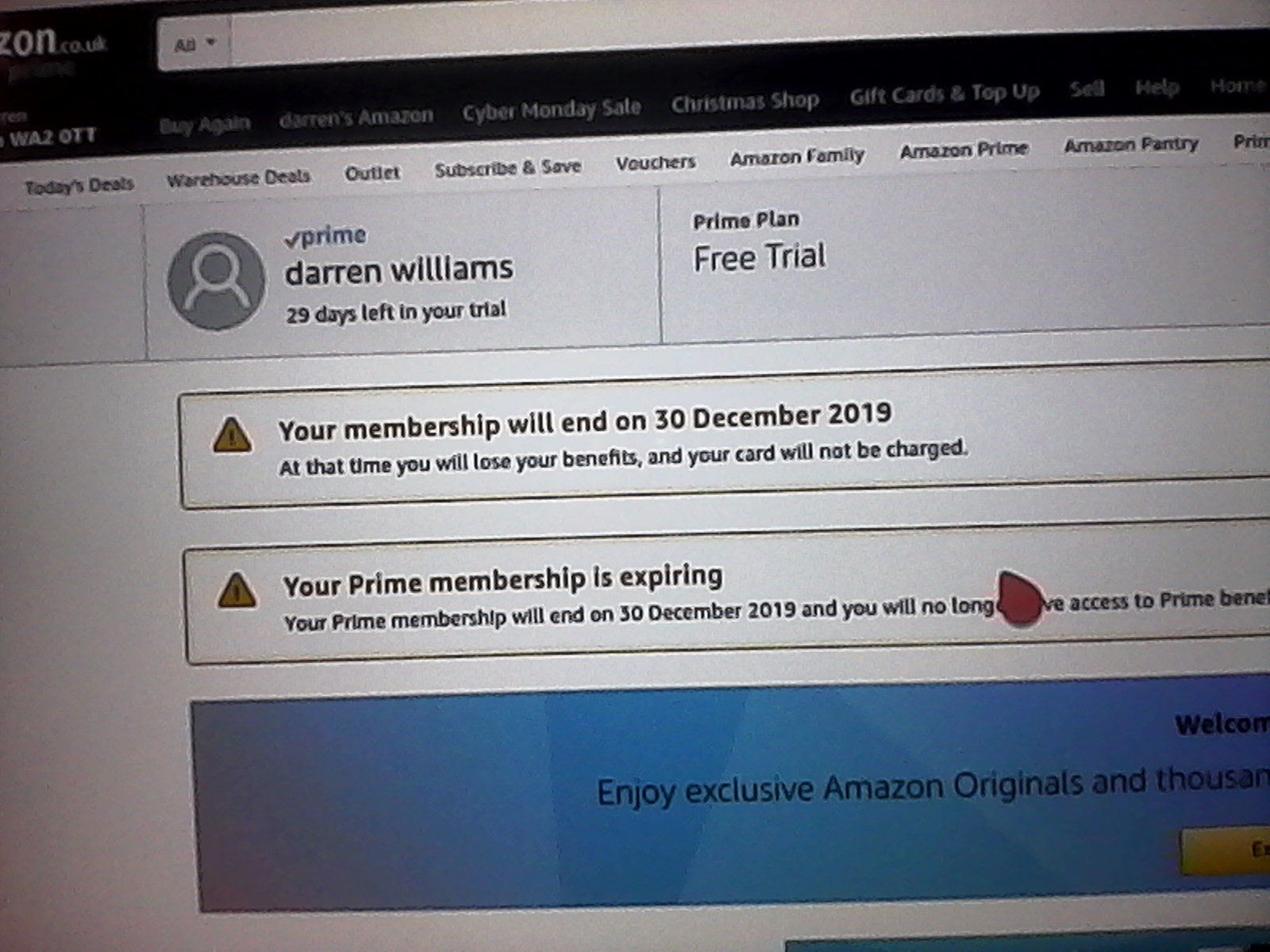This image is a tilted photograph of a section of a monitor displaying the British Amazon webpage (Amazon.co.uk). The top area features several clickable options including "Buy Again," "Darren's Amazon," "Cyber Monday Sale," "Christmas Shop," "Gift Cards & Top Up," "Sell," and "Help." There's also a black bar with options like "Today's Deals," "Warehouse Deals," "Outlet," "Subscribe & Save," "Vouchers," "Family," "Amazon Prime," and "Amazon Pantry." In the middle of the screen, highlighted in various sections and colors, it prominently reads that Darren Williams has 29 days left in his Prime trial. Key details state, "Your membership will end on 30 December 2019. At that time you will lose your benefits and your card will not be charged." Below this is a warning triangle signifying the expiration notice again, reinforcing that the Prime membership will terminate on the stated date, and Darren will no longer have access to Prime benefits. The screen also displays a descriptive section about enjoying exclusive Amazon Originals and other benefits, paired with a yellow button for further actions.